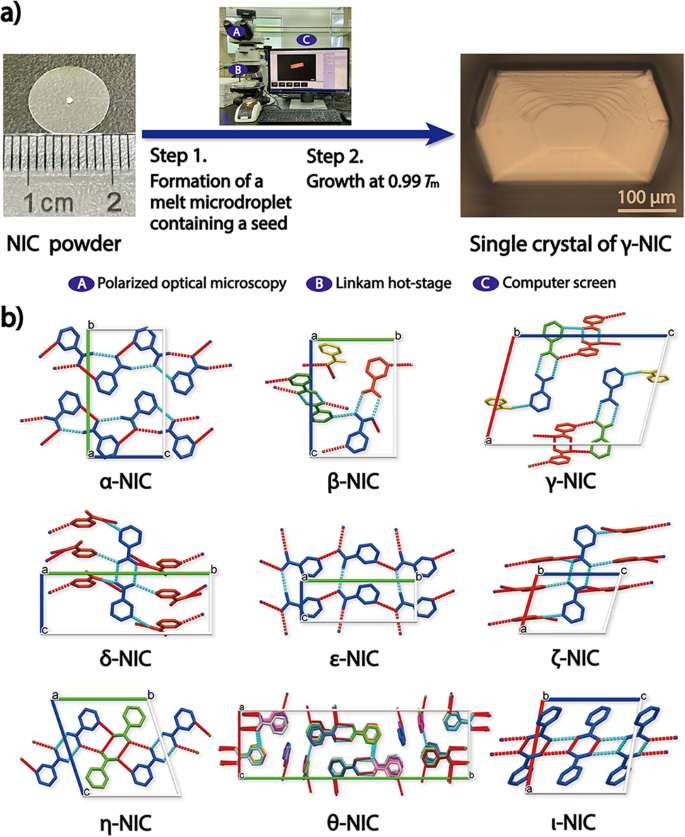The image is a detailed scientific diagram, likely from a textbook, demonstrating the formation and growth of a crystal. The top section, labeled "A," presents three images in sequence. The first image on the left is a close-up shot of a silver, shiny disc, roughly 1 centimeter in diameter, placed above a ruler; this is labeled "NIC Powder." The middle image illustrates Step 1, "Formation of a melt micro-droplet containing a seed," showing what looks like a computer screen. Step 2, "Growth at 0.9 Tm," follows, with an arrow pointing to the rightmost image, depicting a white object labeled as "Single crystal of Y-NIC" with a measurement scale indicating 100 UM. Below this is Section B, containing colorful digital renderings of chemical structures, represented in a 3x3 grid. These molecular images, featuring hexagons and lines in red, green, and blue, detail various stages of chemical compositions, each ending with the capital letters "NIC." The image is clear against a white background and includes text annotations and labels such as "Polarized Optical Microscopy" and "www.cst.eu.com," suggesting microscopic analysis and web resources.